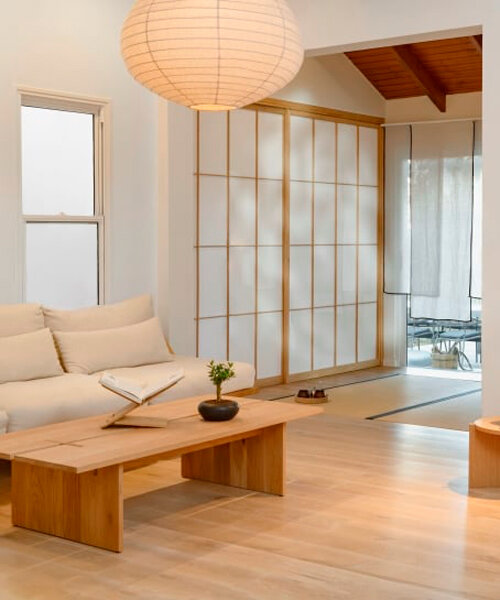This photograph showcases the interior of a serene, Japanese-inspired living room, adorned with a blend of traditional and modern elements. At the forefront, on the left side, is a tan-colored, fluffy futon-style sofa, adorned with matching pillows, and set close to the wooden floor. Adjacent to the low-set sofa, a wooden coffee table hosts a small, vibrant green bonsai plant and an open book on a pedestal, adding a touch of calm and subtle decoration. The background reveals elegant room dividers or shoji screens, and a hint of tatami mat flooring. Above, a large, glowing paper lantern illuminates the space, casting a soft, warm light that complements the muted palette of light pink, beige, and cream tones, which suffuse the room with a light, glowing ambiance. Translucent fabric panels hang gracefully, allowing natural light to gently filter through. A small window on the middle right-hand side offers a glimpse of the sunny day outside, contributing to the room's airy and peaceful atmosphere.